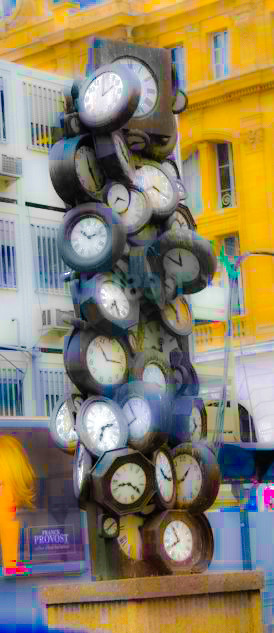This photograph captures an outdoor scene on an overcast day. Dominating the background is a prominent, stone building painted in a striking bright gold hue. The building features several arched windows along its upper floors and rectangular windows on the levels below, adding a touch of architectural elegance. Flanking this structure, we see additional buildings, likely office spaces, distinguished by their more modern windows.

The focal point of the image, however, is a towering and intricate sculpture composed of various clock faces, artfully arranged one atop the other. The clocks are predominantly round, with some unique octagonal shapes integrated into the design. Each clock face is encased in a variety of differently colored and sized frames, contributing to the sculpture's eclectic and captivating appearance. This assemblage of timepieces melds together to form a singular and impressive piece of contemporary art.